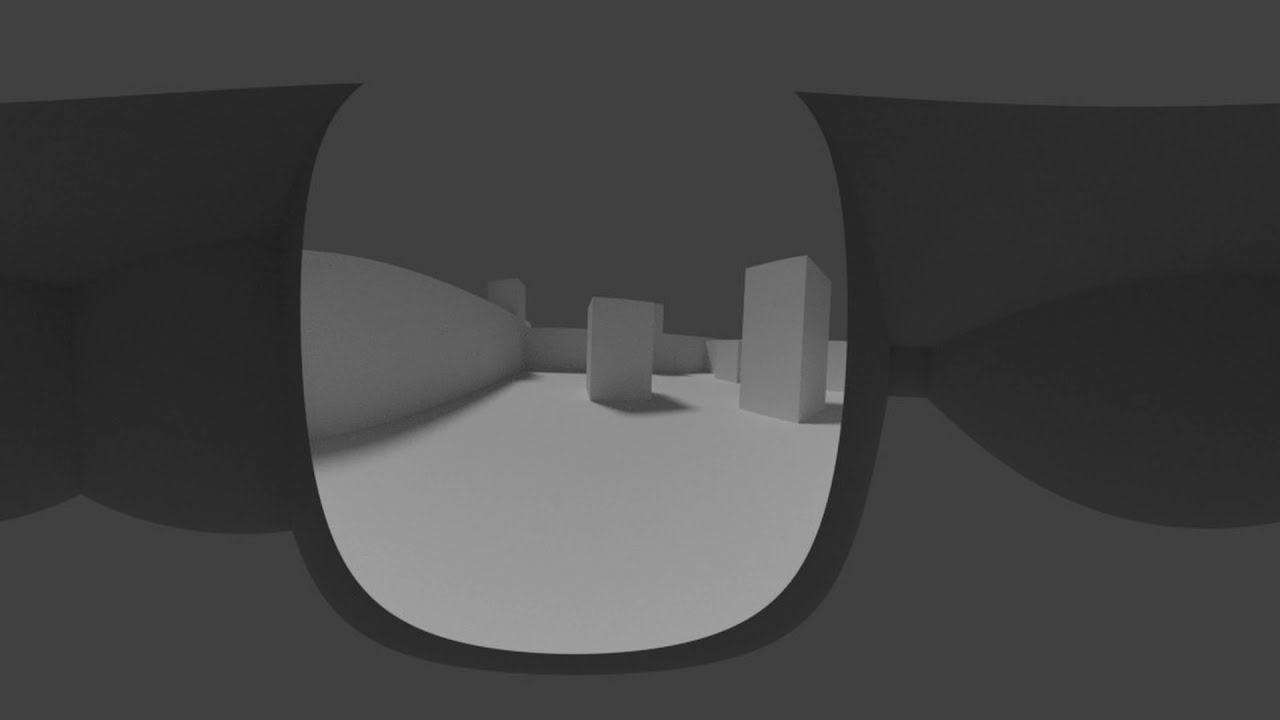The image is a rectangular horizontal illustration featuring a darker color palette of grays and whites. It is bordered by gray sections at the top and bottom. At the left center of the composition lies an oval-shaped graphic, reminiscent of an automobile mirror or a lens of glasses. The view within this oval displays an abstracted, upper-patio area with concrete flooring, walls, and a couple of rectangular structures casting distinct shadows. The setting inside the lens appears to be a stark, minimalist cityscape with plain white blocks representing buildings, against a gray-scale background. Outside the lens, the image transitions back to the gray-toned surroundings, suggestive of the rims of glasses, accentuating the monochromatic contrast and abstraction within the artwork.